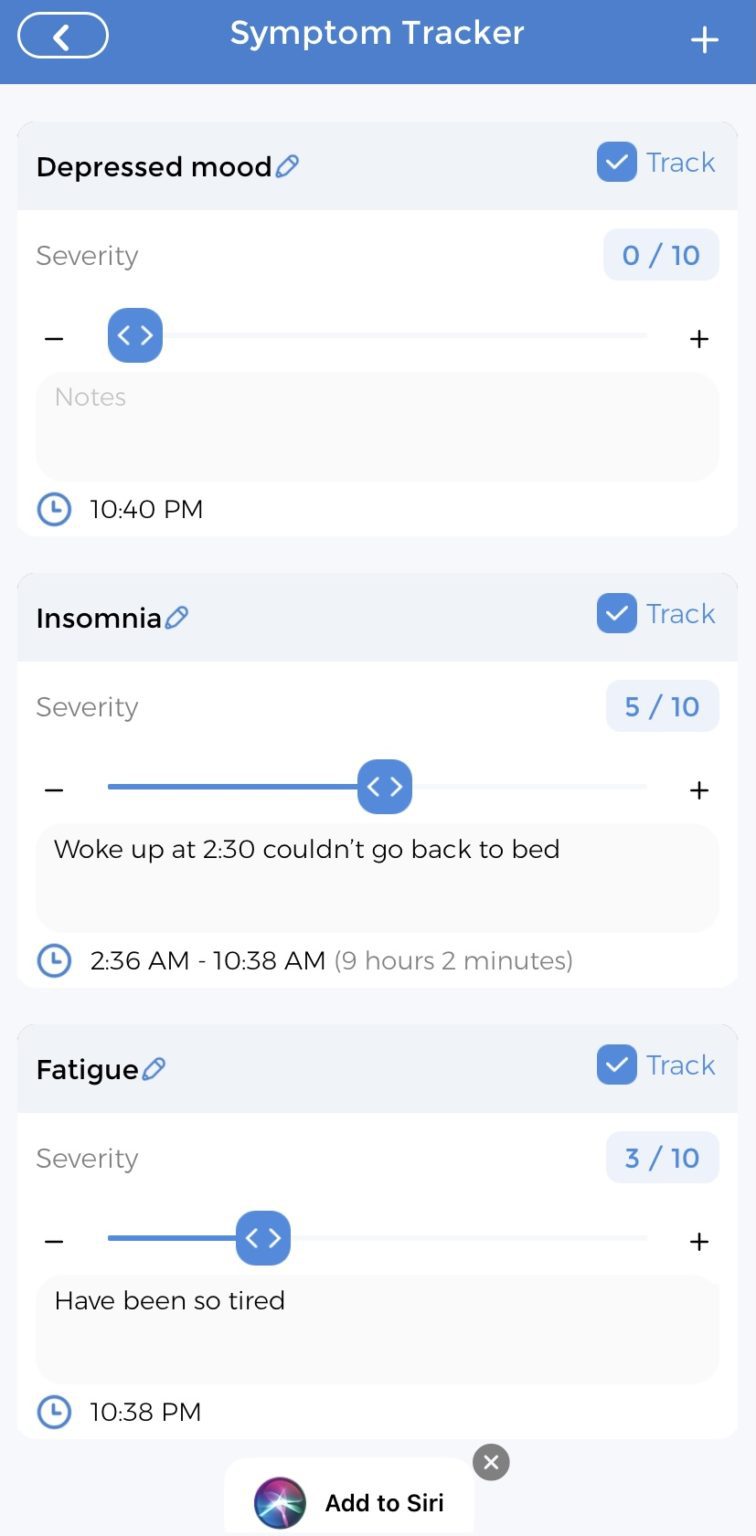This screenshot features a detailed view of the Symptom Tracker app interface, presenting user-reported symptoms and their respective severities. 

At the top, a blue banner stretches across the width of the screen. On the left side of this banner, a white oval-shaped icon with an accompanying arrow is displayed. Centrally positioned in bold, white text, the words "Symptom Tracker" stand out, written with capitalized 'S' and 'T,' and sized slightly larger than the surrounding text. To the right, a plus sign is visible within the banner.

Below this section, the background transitions from light to dark gray, highlighting distinct symptom entries. The first entry reads "Depressed Mood" in black text with a capital 'D' next to a blue pencil icon. A blue square with a white check mark and the word "Track" (capital 'T') is aligned to the right. 

Following this, set against a white background, the label "Severity" is displayed with "0/10" next to it and an accompanying slider for user input. Below this, the text "Notes" appears near a clock icon indicating "10:40 p.m." The second symptom listed is "Insomnia," with a similarly styled blue square and check mark, next to the 'Track' option. The severity is shown as "5/10" with the slider positioned accordingly. User notes include: "Woke up at 2:30. Couldn't go back to sleep. Back to bed."

The user’s sleep duration is recorded as "2:36 a.m. to 10:38 a.m.," totaling "9 hours 2 minutes." Another symptom "Fatigue" is presented with 'Track' and a severity rating of "3/10." A note reads: "Have been so tired." Timestamped at "10:38 p.m.," it ensures precision in reporting.

At the bottom of the screen, "At Siri" is noted with a little circle containing an 'X' to the right, possibly functioning as an interaction option.